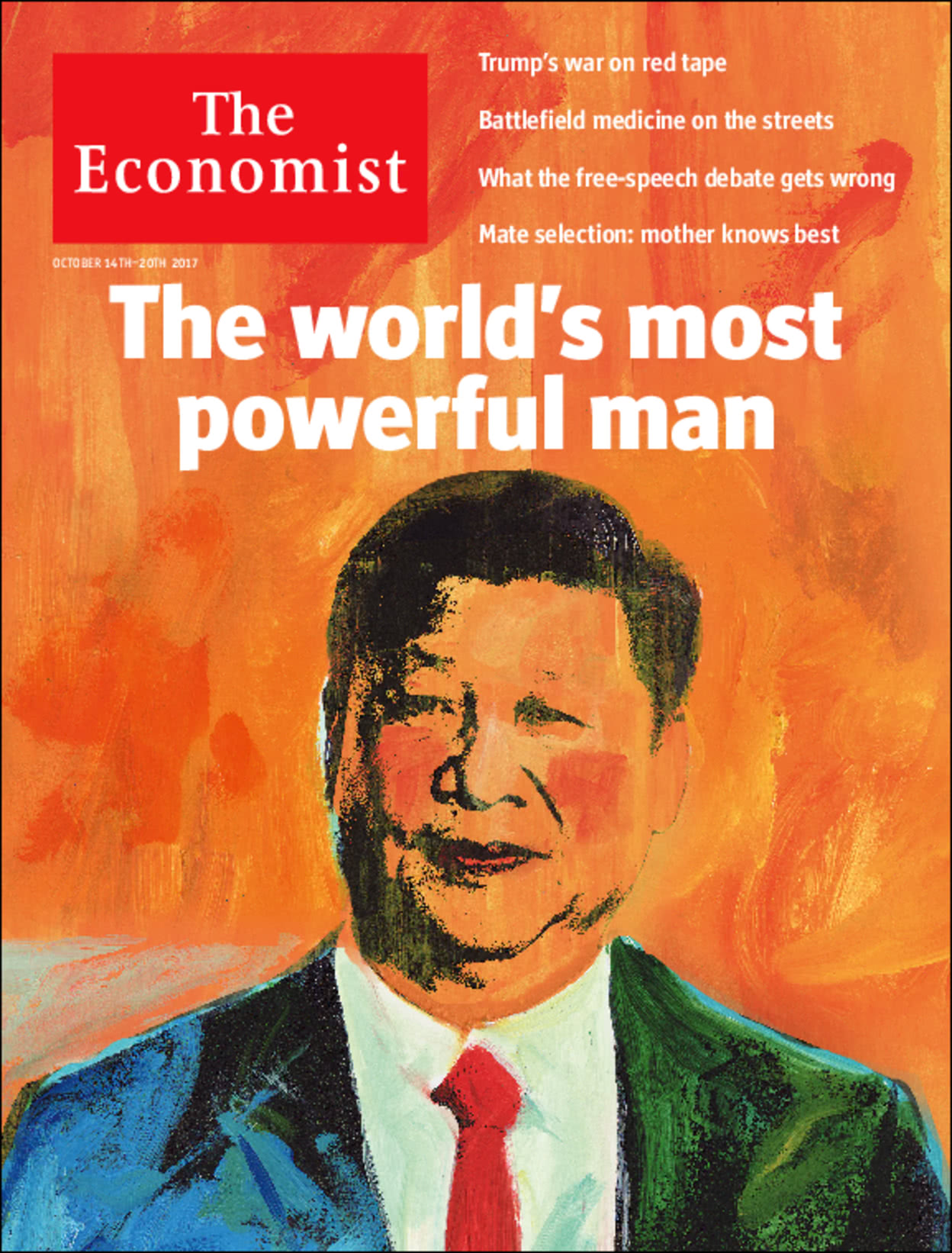This is a detailed and descriptive caption for the magazine cover featuring an illustration of Chinese President Xi Jinping:

"The cover of the October 14th to 20th, 2017 issue of The Economist features a hand-drawn image of what appears to be President Xi Jinping of China, though some details suggest it may not be an exact likeness. Xi is depicted with black hair, pink cheeks, and a clean-shaven face, wearing a suit jacket with blue shading on the left side and green shading on the right, paired with a red tie and a white button-down collared shirt. Dominating the cover is the headline, 'The World's Most Powerful Man,' likely referring to Xi Jinping. The background of the cover is an orange and red gradient, reminiscent of the Chinese Communist Party's official colors. The masthead reads 'The Economist' in white lettering within a reddish-orange rectangle. Four secondary articles are advertised: 'Trump's war on red tape,' 'Battlefield medicine on the streets,' 'What the free speech debate gets wrong,' and 'Mate selection: mother knows best.'"